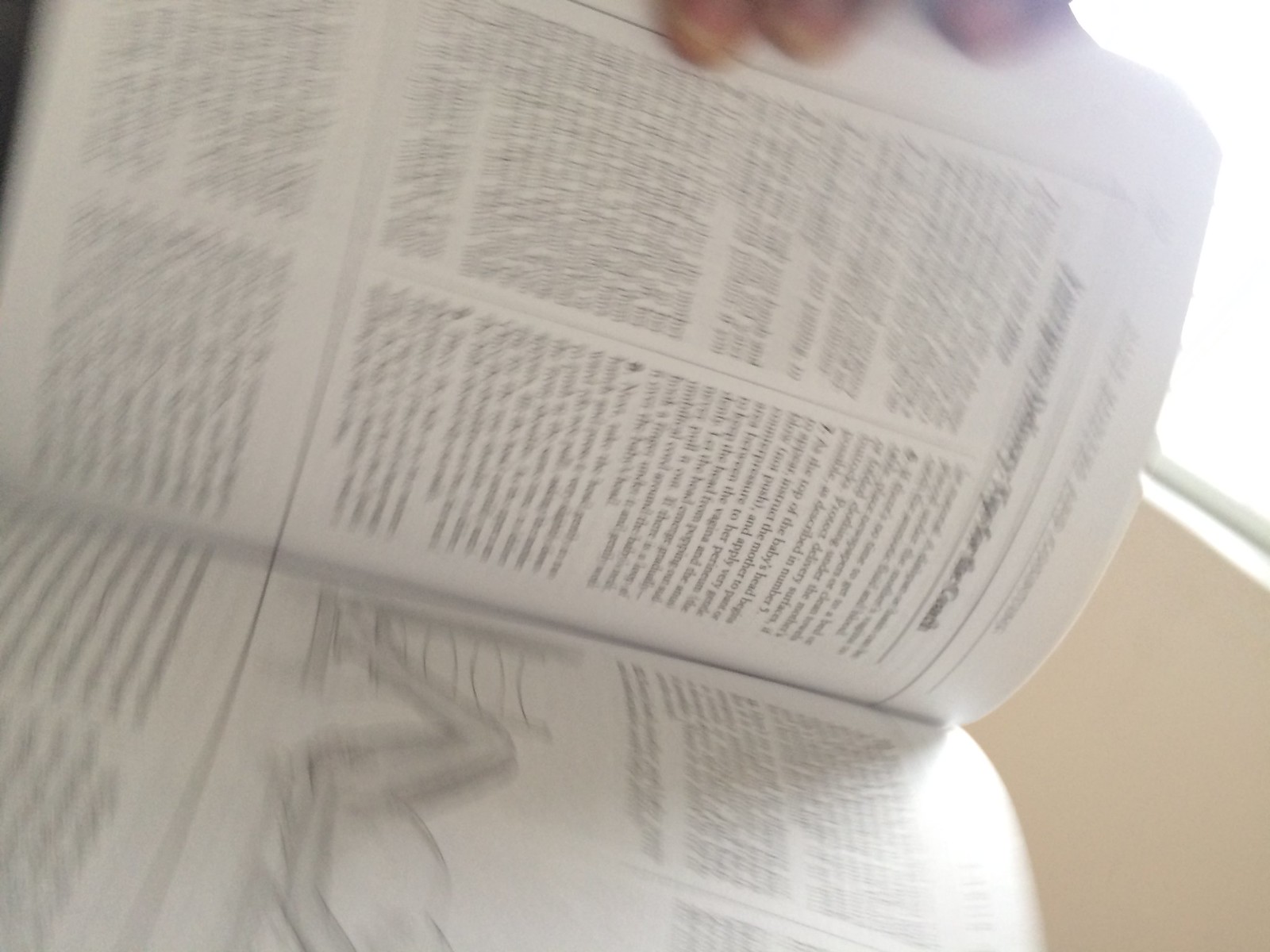The photograph captures a blurry image of an open book, held open by a hand visible at the top of the frame. Despite the lack of clarity in the text, the book appears to feature a pen and ink drawing that showcases a specific posture. The illustration depicts an individual lying or reclining on a surface with their knees bent and raised in the air, suggesting either a yoga pose or an instructional depiction related to childbirth. The person's profile hints at pregnancy, but the blurriness makes it challenging to determine the exact nature of the demonstration. Light from a nearby window illuminates the scene from the right side, casting a soft glow on an off-white wall in the background. Multiple fingers are seen holding the book open, providing a closer view of this intriguing, yet ambiguous illustration.